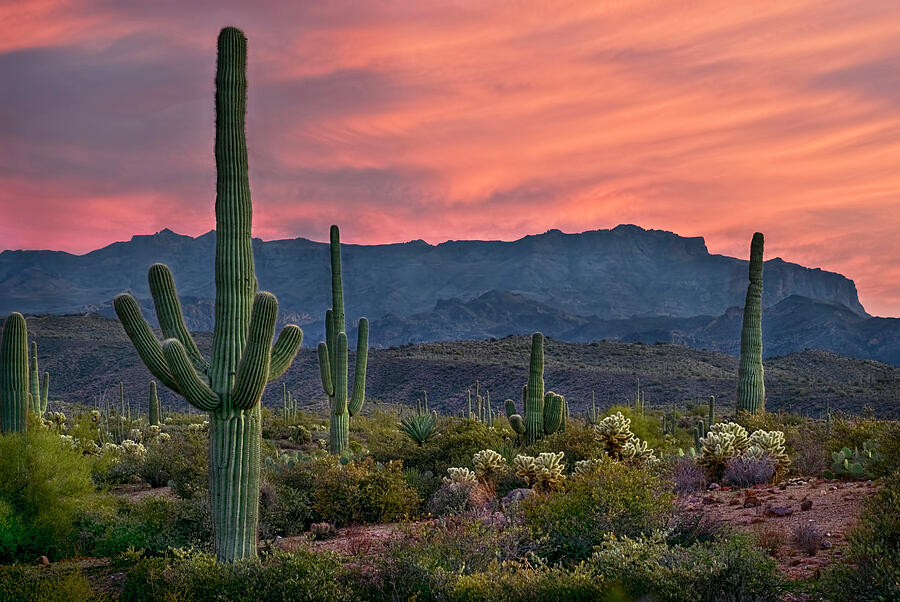The image depicts a high desert landscape featuring numerous healthy saguaro cacti. Dominating the foreground on the left side is a towering saguaro, approximately 15 feet tall, with one central stalk and five arms radiating from its lower part. This imposing cactus contrasts with a smaller, arm-less saguaro in the middle distance. The ground around the cacti is dotted with various green, brown, and light green bushes, some of which bear white blooms, as well as scrub brush and rocks. In the background, a series of low, craggy hills rise to meet a taller hill, ultimately leading to a distant mountain ridge. The sky, occupying nearly half of the upper portion of the image, transitions from blue on the left to pink on the right. Wispy gray clouds float against the gradient, suggesting the time is either dawn or dusk.